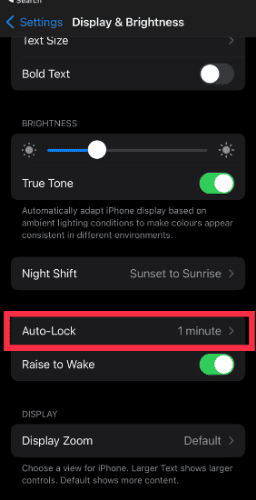The image depicts a smartphone interface featuring a dark-themed "Settings" menu. At the top left, the word "Settings" is highlighted in blue. Below, the section titled "Display & Brightness" appears in white.

The page is divided into multiple sections, each enclosed in boxes:

1. **Text Size**: The header "Text Size" is in white, accompanied by a right-facing arrow on the right-hand side.
2. **Bold Text**: This section displays a toggle button, which is currently off.

The next section deals with screen brightness:
1. **Brightness**: Within a box, there is a sun icon on both the left and right sides, flanking a blue bar that represents the brightness level. A white dot on the bar shows the current position, which is slightly towards the left.
2. **True Tone**: This feature is listed below, along with an explanation: "Automatically adapt iPhone display based on ambient lighting conditions to make colors appear consistent in different environments." The toggle button for this feature is green and turned on.

Further down:
1. **Night Shift**: Indicated in white text, states "Sunset to Sunrise."
2. **Auto-Lock**: Displayed with "1 Minute" enclosed in a red border.

At the bottom, additional settings include:
1. **Raise to Wake**: This feature is enabled, indicated by a green toggle button.
2. **Display Zoom**: The section reads "Display Zoom: Default," with instructions that selecting "Larger Text" shows larger controls while "Default" displays more content.

This comprehensive and well-organized layout allows easy navigation and adjustment of display and brightness settings on the device.